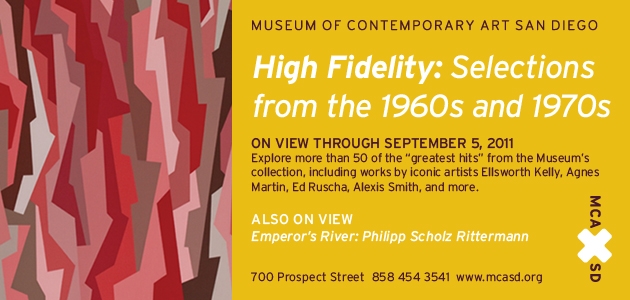The advertisement poster from the Museum of Contemporary Art, San Diego, features a striking gold background where the text is situated. On the left side, there is an artistic graphic with striations in light pink, red, gray, brown, and beige, descending downwards. The right side of the poster highlights in bold, white text: "High Fidelity Selections from the 1960s and 1970s," which is on view through September 5, 2011. The exhibition invites visitors to explore more than 50 of the greatest hits from the museum's collection, showcasing works by iconic artists such as Ellsworth Kelly, Agnes Martin, Ed Ruscha, Alexis Smith, and more. Additionally, the poster promotes another exhibition titled "Emperor's River" by Philip Schultz Ritterman. At the bottom, crucial information is provided in brown text, including the address: 700 Prospect Street, phone number: 858-454-3541, and website: www.mcasd.org.